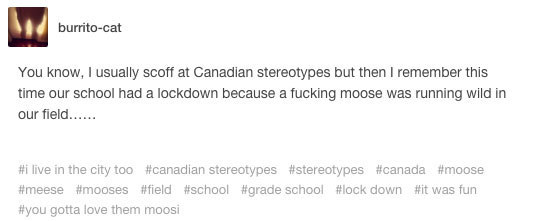The image consists primarily of text set against a plain white background, with the overall quality being quite poor—blurry and fuzzy. In the top left corner, there is a small, indistinguishable piece of artwork in black and white. 

To the right of the artwork, the text reads "Burrito-Cat." Beneath that, the text narrates, "You know, I usually scoff at Canadian stereotypes, but then I remembered this time our school had a lockdown because a F-U-C-K-I-N-G moose was running wild in our field...."

Following this anecdote, several hashtags are listed: 
- #ILiveInTheCityToo
- #CanadianStereotypes
- #Stereotypes
- #Canada
- #Moose
- #Meese (spelled M-E-E-S-E)
- #Moosehead